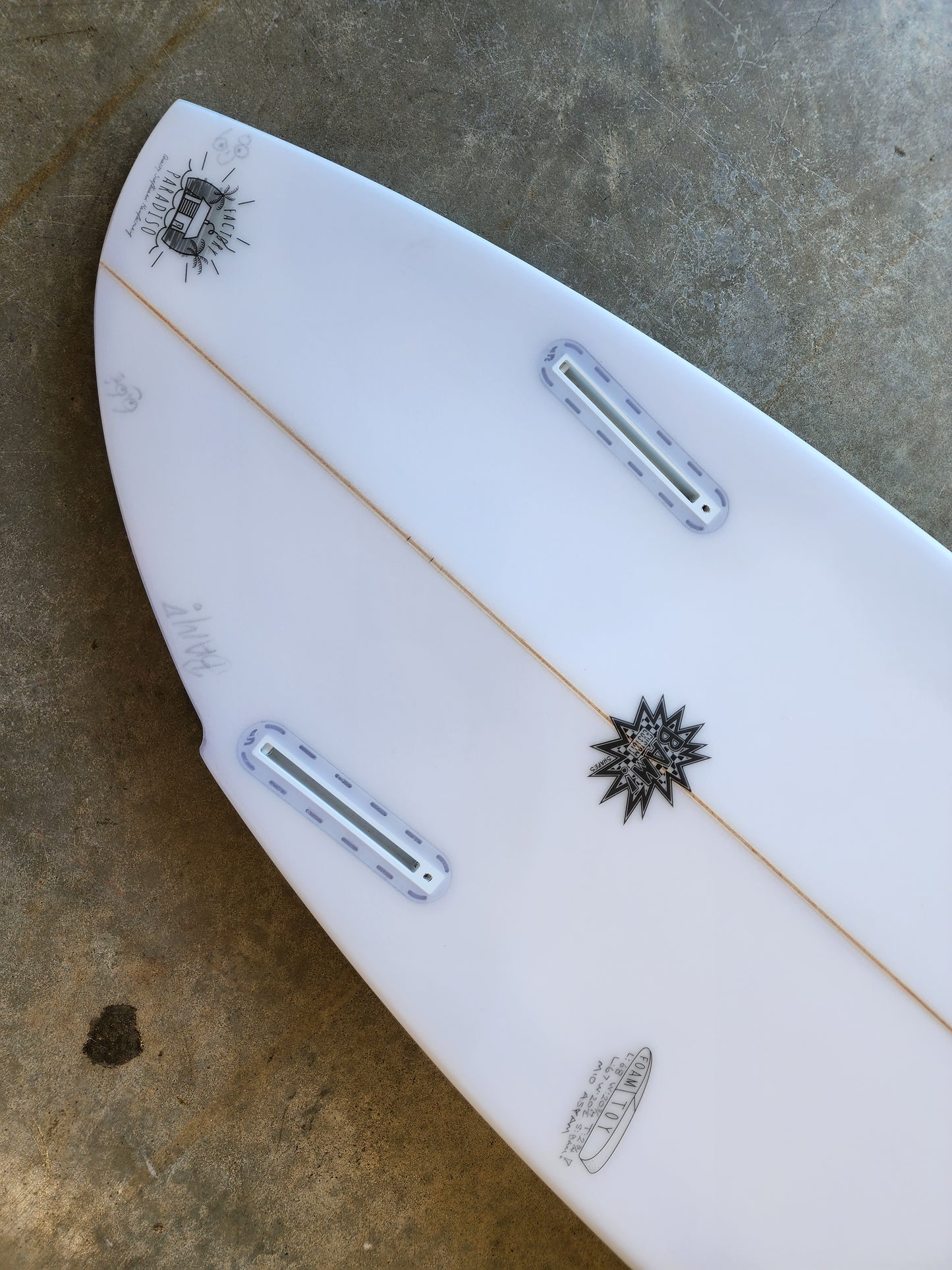The photograph, vertically-oriented, captures an all-white, long plastic or composite fiberglass object that closely resembles a surfboard or sailboard, resting on a dirty concrete surface. The board is marked by an orange seam running down its center and features two narrow slots: one on the lower left and another on the upper right. A striking sticker positioned centrally on the board depicts a dramatic, comic-style "BAM" with lines jutting out to emphasize its impact, alongside the words "Foam Toy" and an 'M!' on the left in grey, which is not another sticker. Additionally, a small black star-like sticker intersects the seam in the middle of the board. The concrete below is notably grimy, with an old, dried, blackened piece of gum visible to the left. Despite the lack of size reference, the photo strongly suggests the item is designed for water or perhaps as part of a child's toy plane.